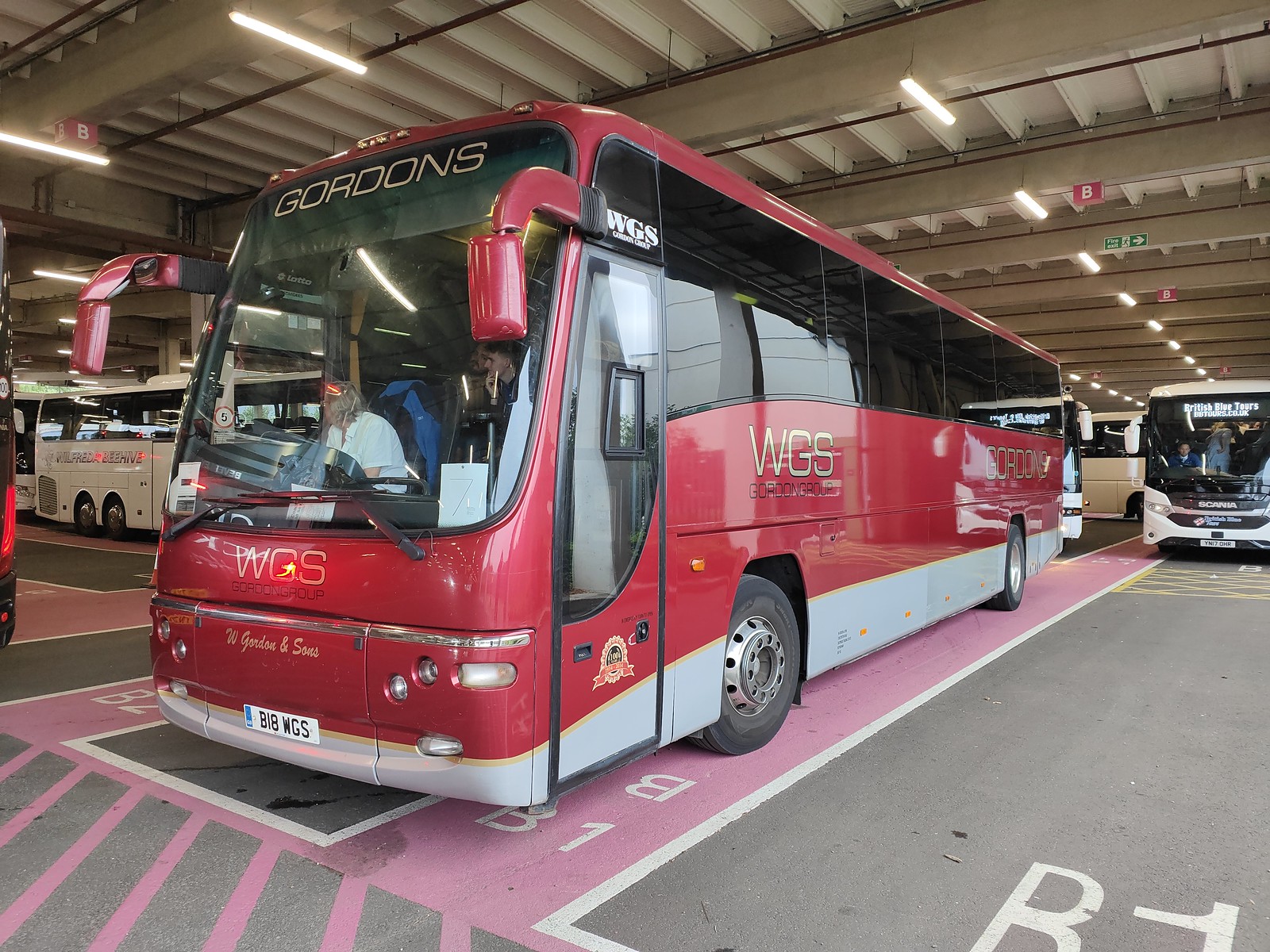This daytime photo captures a busy parking garage, likely a bus depot, filled with several modern buses. The focal point is a striking red bus, almost maroon in color, featuring the name "Gordon's" prominently displayed on a black-tinted glass area at the top. This bus, marked with a B2 designation on the gray and pink striped flooring, also has a large front window and a light gray stripe along its bottom, while its side windows are tinted in black. The driver's clear window reveals the driver seated in the front, while one passenger inside rests his hand on his chin. Surrounding the red bus are additional buses, primarily white in color, and equally modern in design. One white bus in the background shows a driver wearing a blue shirt over a white t-shirt. The garage's open structure reveals bolted light fixtures and hanging wires, adding to the industrious atmosphere. Reflections on the shiny red bus and the organized parking slots emphasize the orderly arrangement within the garage.